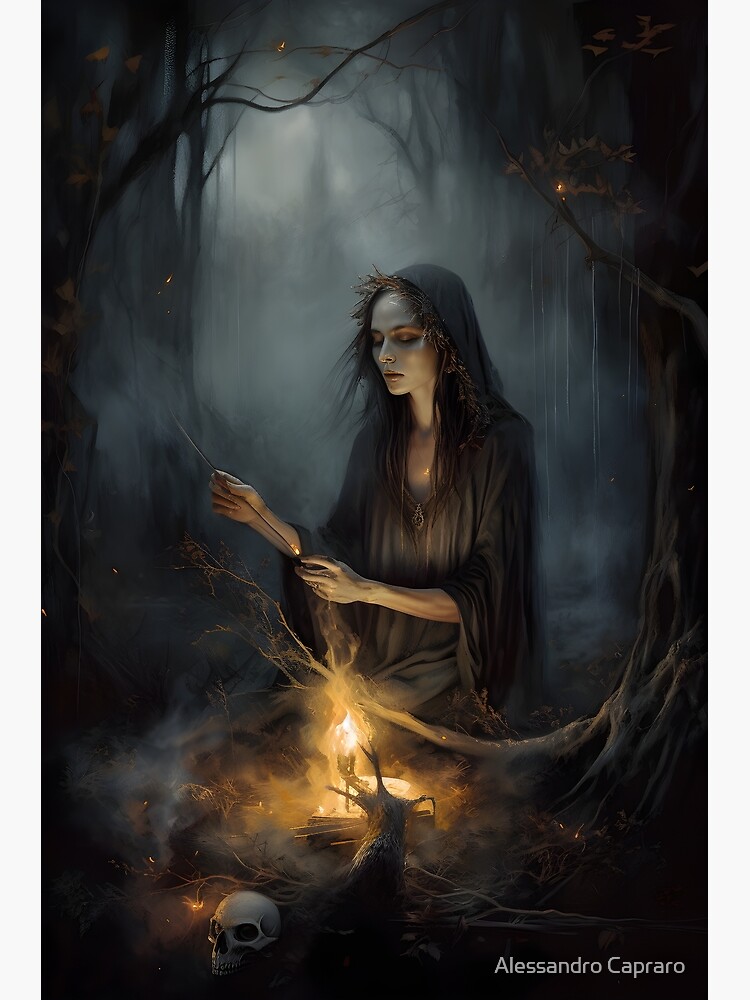In a dark, moody, and stylized color illustration reminiscent of video game art or a book cover, a central, witch-like female figure commands attention. Kneeling on the ground and facing left, she is draped in a long hooded black cloak that shrouds her dark hair and pale skin, adding to her enigmatic presence. Her eyes are closed or lowered, intensifying the air of concentration as she holds a burning ember in her hands. Below her, an eerie fire—resembling a nerve cell ganglion or twisted tree roots—burns, casting a spectral glow. The background reveals a mystical forest, shrouded in fog and mist, with smoky, blurred trees arching over her. Surrounding her are twigs, branches, and a skull lying in the bottom left corner, contributing to the arcane atmosphere. The name "Alessandro Caprero" is subtly inscribed in light gray in the bottom right corner, anchoring this haunting and magical scene.